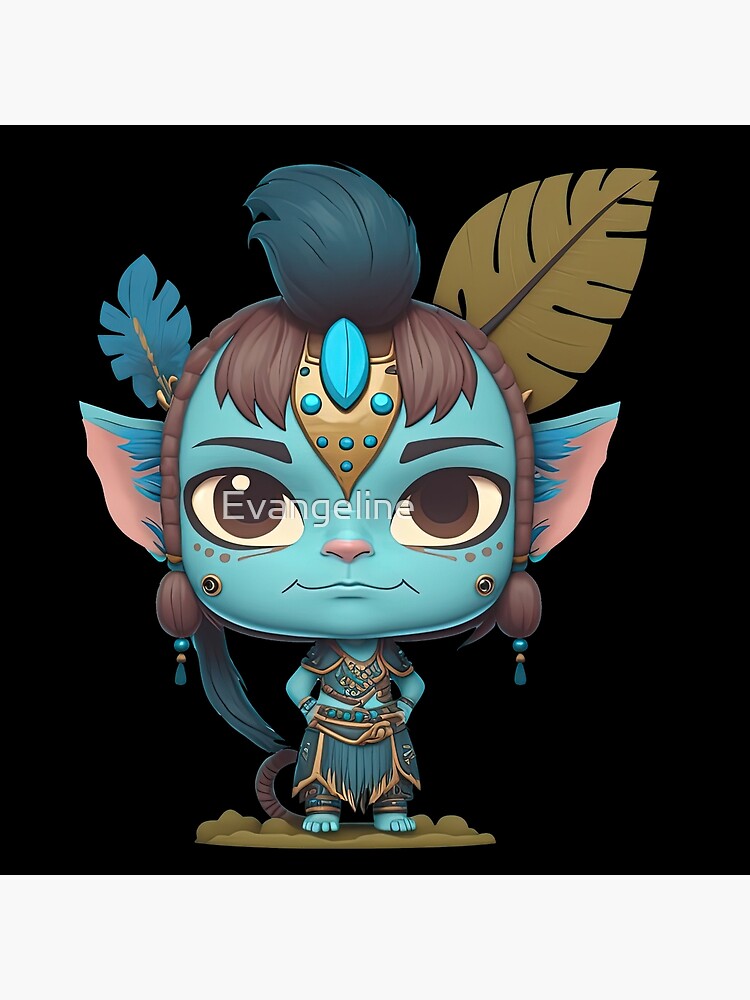The image depicts a digital painting of a small, mythical blue character with features reminiscent of a Funko Pop figurine and elements inspired by the characters from Avatar. The character has a disproportionately large, rounded square head and a much smaller body. Its skin is blue, and its face features large, expressive brown eyes, a small flat nose with a pink tip, and a thinly drawn mouth in black.

A black and gold, triangular headpiece adorned with turquoise and jade jewelry extends from the forehead to the nose. The character's hair is brown with two braids on the sides and a tuft of blue hair in front of the headpiece. The ears are pointed and blue with pink inner edges. There are two feathers at the back of the character's head—a smaller blue feather and a larger golden leaf-like feather.

The character wears a tribal warrior-like outfit with black and gold accents, and stands with bare blue feet on a small brown platform that has a light beige-tan hue. A blue tail can be seen curling behind the character. The background is entirely black, and the name "Evangeline" is written across the character's face.